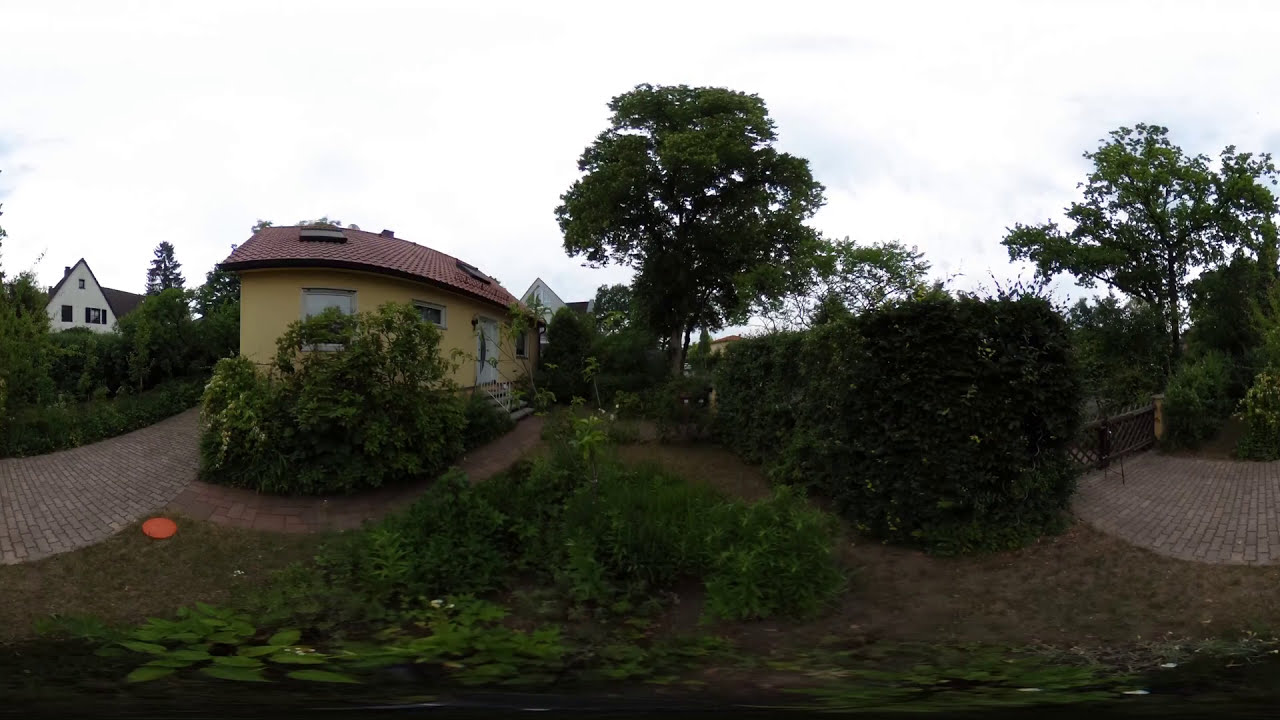This photograph captures a quaint, outdoor garden scene on a cloudy day, likely in Britain. The image is wide and somewhat panoramic, slightly distorted in the manner of such shots. The foreground is filled with green grass, bushes, and shrubs, with a cobblestone brick path winding through the scene. On the left, a simplistic, yellow house with a red tile roof stands out, with white stairs leading to its front door. Directly to the left, partially obscured by trees and shrubs, a white two-story house with a triangular pointed roof peeks out. The right side features a tall shrub fence and another brick path curving around a tree and circling a patch of ground. The sky overhead is light gray, with patches of white clouds diffusing the daylight, casting soft shadows over the landscaped garden dotted with green trees and plants. There is a suggestion of a pond further down, although it is not clearly visible. The overall serene environment evokes a feeling of tranquil English countryside.